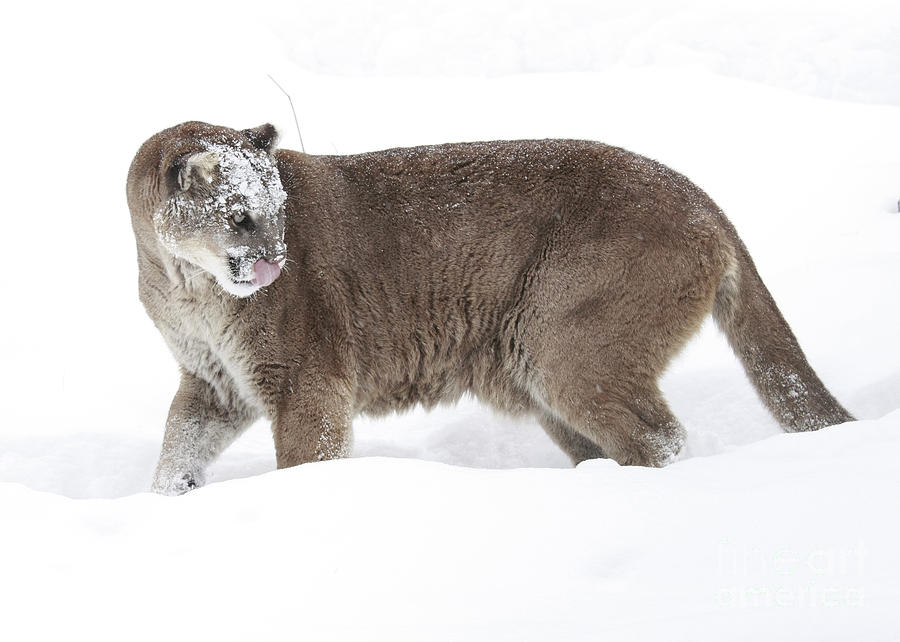The image captures a large cougar, also known as a mountain lion, in a snowy landscape, with its body facing left and its head turned to the right. The cougar's dark brown fur is contrasted by the white snow all around, with snowflakes visible on its face, particularly around its forehead, eyes, and nose. The cat's pink tongue sticks out in a circular motion, licking snow off its nose. The snow reaches up to the cougar's ankles, covering parts of its tail and the ends of its feet. The animal's side profile reveals its front leg positioned ahead of the other, while its back legs appear parallel. The cougar’s underbelly has lighter brown fur, and its mouth has a hint of black coloration. The dense snow, reflecting light, makes its features stand out distinctly, especially in the shaded areas. The scene suggests a possible hunting scenario, and hints at a mountainous region, possibly on the West Coast of the United States.